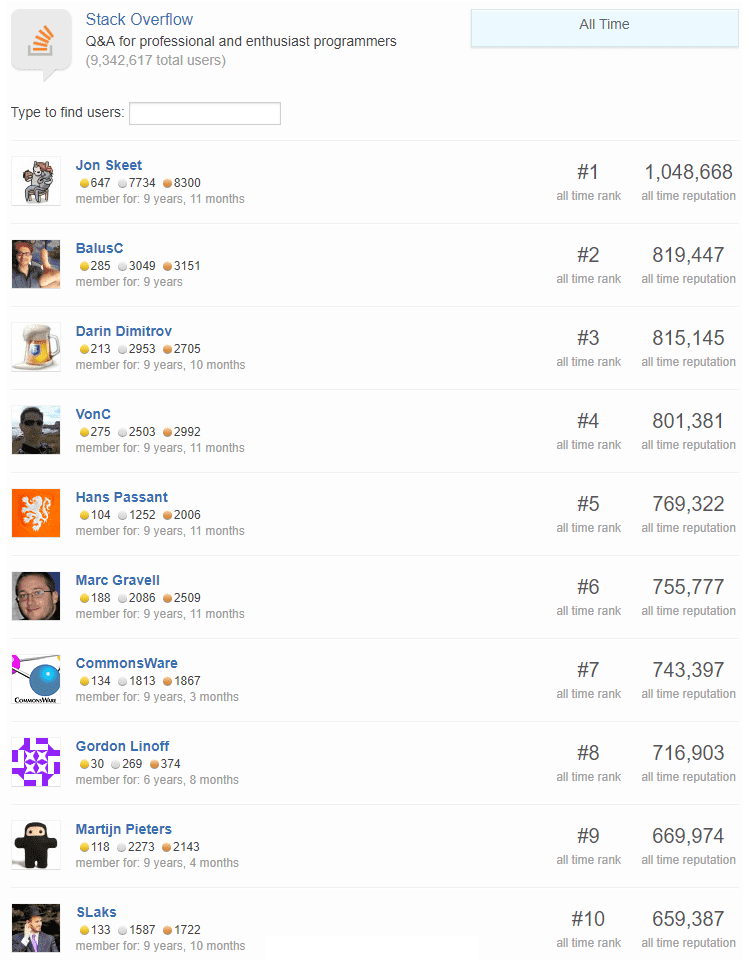The image features a page from Stack Overflow, the popular Q&A platform for professional and enthusiast programmers. The page shows a ranking of the top contributors based on their reputation scores, which they have earned by providing helpful and accurate answers to user questions. 

At the pinnacle of this ranking is Jon Skeet, boasting an unparalleled reputation score of over one million. His profile shows that he has accumulated more than 8,000 bronze badges, 650 gold badges, and numerous silver badges. Following Jon Skeet is a list of other high-ranking members like BalusC and others, each highlighted with their impressive reputation scores and badge counts. 

The ranking continues down to the 10th position, occupied by a user named "SSlacks," who has achieved a reputation score of 660,000. Most of these top contributors have been active on the site for around nine years, signifying their long-term dedication and significant impact on the Stack Overflow community. 

The badges under each user’s name—gold, silver, and bronze—serve as visual representations of their specialized contributions and expertise in the community.